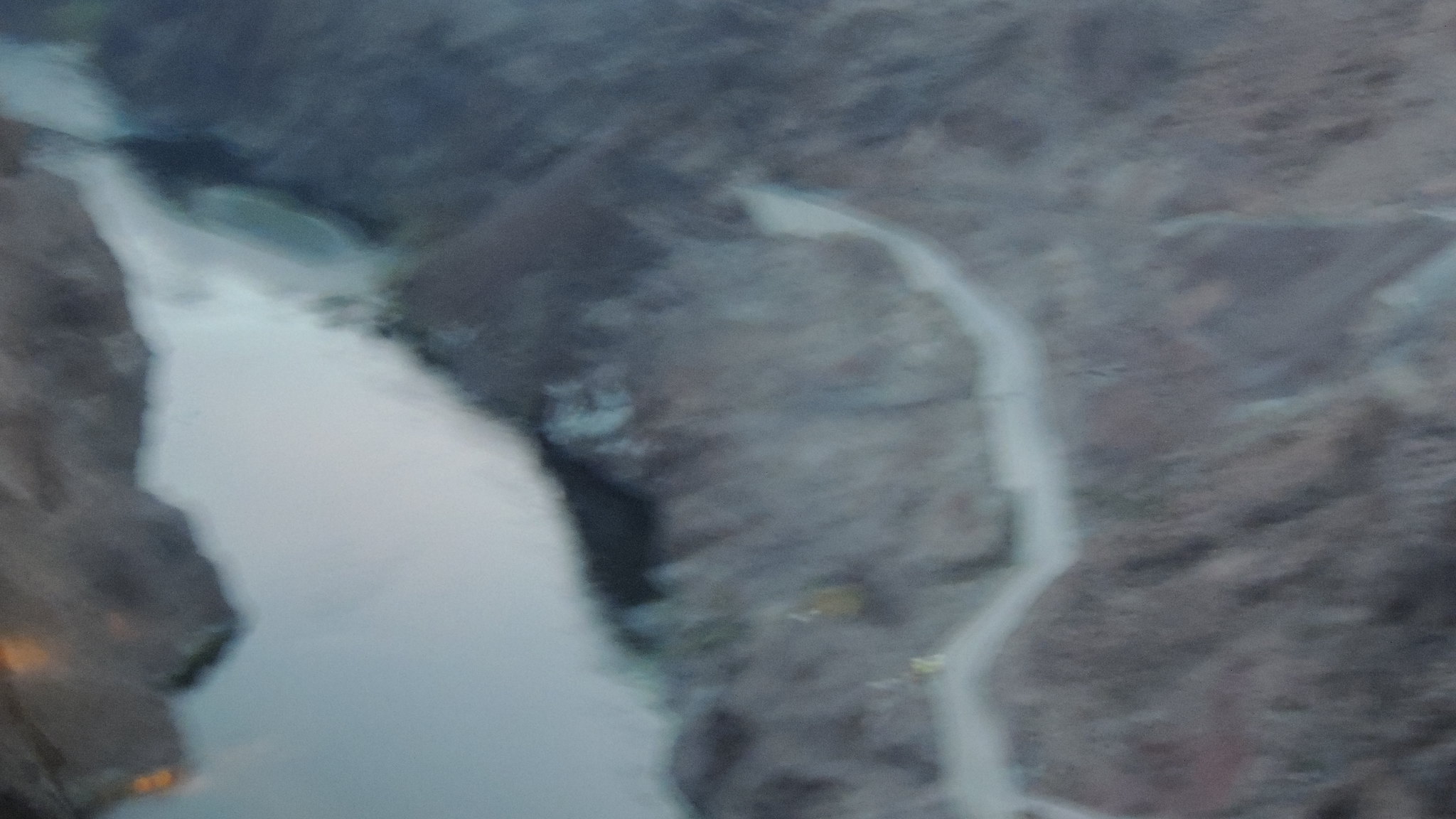This blurry landscape photograph, taken in a landscape aspect ratio, appears to capture an outdoor scene at dusk. The image is marred by significant motion blur, likely due to camera shake, making discrete details difficult to discern. Dominating the right two-thirds of the frame is a rugged rocky outcropping, primarily gray with subtle reddish undertones. A road runs along the base of this rocky formation. To the left of the outcropping lies a body of water, possibly a river, flanked on its opposite shore by more rocky terrain. The horizon is not visible in this image, emphasizing the immediate landscape rather than the broader surroundings.